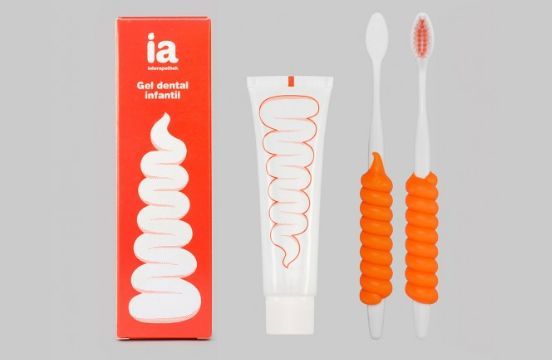This advertisement features a dental care set aimed at children, comprising a toothpaste tube, toothbrushes, and their packaging. The background is a plain gray, contrasting sharply with the vibrant orange and white color scheme of the products. On the left side of the image is an orange box labeled "IA Gel Dental Infantil," adorned with a whimsical, whipped cream-like swirl of toothpaste. Adjacent to this is a white toothpaste tube with the same orange-bordered swirl design and a white cap. To the right of the toothpaste, two toothbrushes are displayed, one facing forward and the other backward. Both toothbrushes are primarily white with orange bristles, featuring an orange swirl design that wraps around their handles, adding a playful touch.